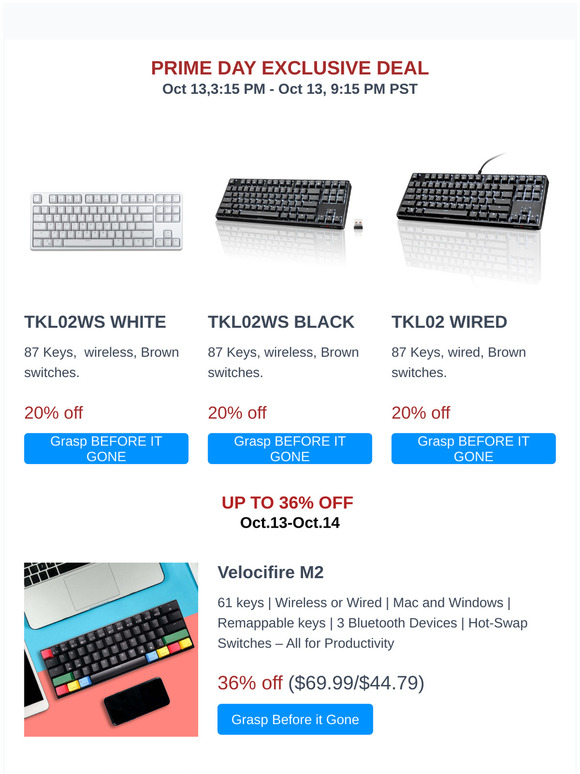The image features a promotional banner for a "Prime Day Exclusive Deal" on various keyboards. At the top, a light gray banner spans the width of the image, with the promotional text in bold red, "Prime Day Exclusive Deal." Below, important timing details are highlighted in black text, stating, "October 13th 3:15 p.m. to October 13th 9:15 p.m. PST."

On the right side of the image, there is a white keyboard labeled "TKL02WS White" with 87 keys and wireless brown switches. A red text below this label offers a 20% discount. Further emphasis is given with a blue rectangle featuring white text that reads, "Grasp Before It's Gone."

Center stage, two additional keyboards catch the eye - both black. The middle keyboard is also labeled "TKL02WS Black" with 87 keys and wireless brown switches. Similarly, it is marked with a "20% off" discount in red text, and the blue rectangle with "Grasp Before It's Gone" in white text repeats this urgency.

The bottom section of the image displays another black keyboard, notable for its colorful keys: a mix of red, green, blue, and yellow. Below this keyboard, a black smartphone with a blank screen is partially visible, adding a modern touch to the composition. 

Overall, the image is a visually engaging promotion, drawing attention to the exclusive Prime Day deals with clear, colorful, and detailed descriptions of the featured keyboards.